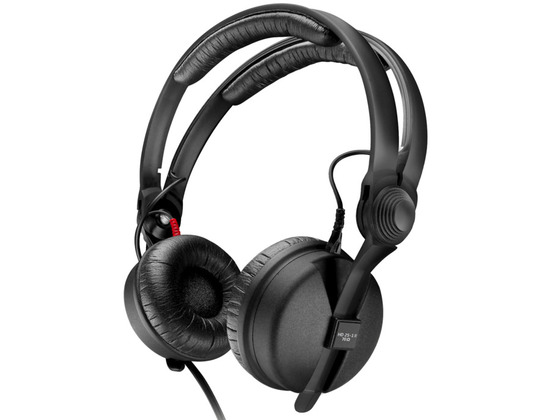This image features a sleek pair of black headphones set against a plain white background. The headphones are detailed with substantial cushioning on both the ear cups and the top headband, ensuring a comfortable fit over the head and ears. The headband consists of two arched black bars connected by dual cushions at the top. These ear cups resemble winter earmuffs and are likely made of black leather or a similar fabric, enhancing their comfort. Black plastic pieces connect the headphones to the headband, while wires extend from each ear cup to the top part of the headband. An additional wire protrudes downward from the left side, presumably for connecting to an audio device. On the outer part of the right ear cup, there is a barely legible square label. The minimalistic white background emphasizes the headphones, making this image ideal for a product showcase.